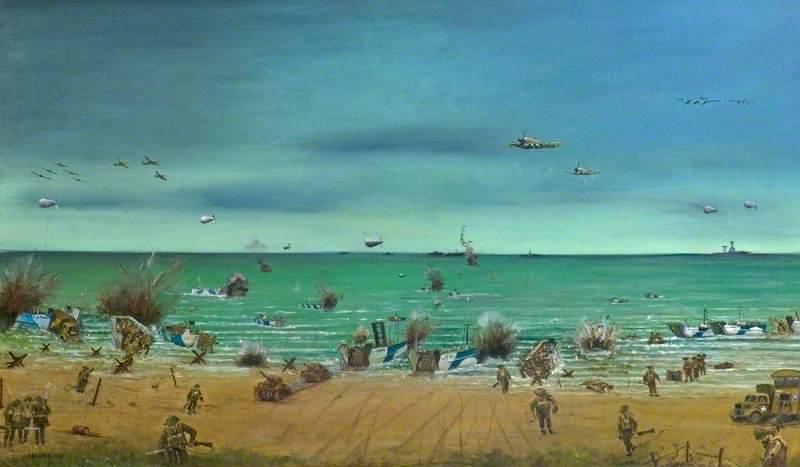This detailed hand-drawn painting captures a dynamic World War II-era military action on a beach, likely inspired by the D-Day invasion. The vibrant teal blue sky dominates the top half of the frame, filled with various aircraft, including fighter jets, bombers, and a Zeppelin centered just above the horizon. On the horizon line, several warships are visible, with a prominent large warship on the right and smaller distant ones in the center.

The middle third of the frame showcases teal green waters dotted with blue and white striped boats, many trailing puffs of smoke as they head toward the central beach area. Closer to the shore, larger boats, also emitting smoke, are unloading troops. The sandy, gold-colored beach itself, marked with tire tracks, features numerous soldiers wearing wide green helmets and matching military uniforms, all carrying rifles. They are seen moving to and from the boats amidst the chaos of war.

The beach is scattered with metal cowl traps and motor vehicles, including a truck on the right marked with a white star. At the very bottom of the frame, a line of grass is visible, and in the bottom right corner, a figure with a megaphone overlooks the scene, possibly directing the troops.

The painting also contains a dark, somber atmosphere with explosions and smoke indicating the violent nature of the battle. The scene overall evokes a sense of urgency and tragedy, depicting injured and fallen soldiers, and the stark realities of war.